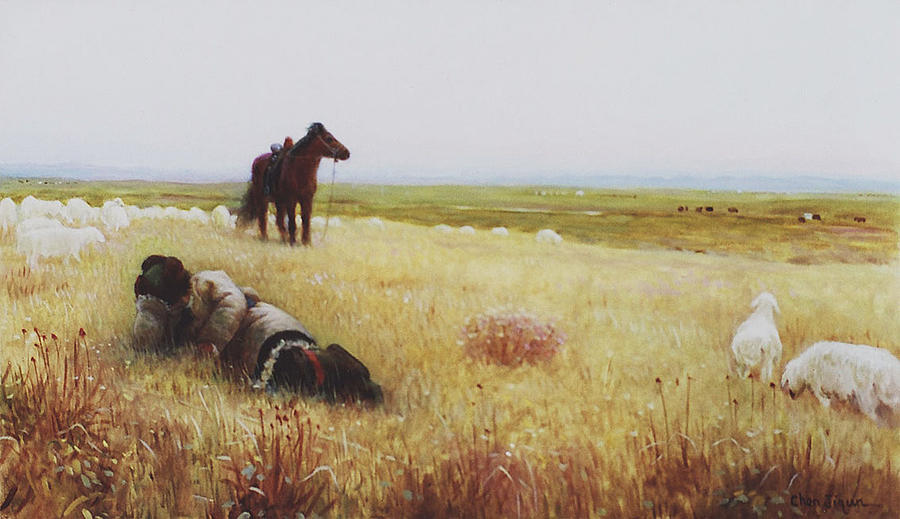The painting depicts a serene rural scene featuring a vast, open field with tall, yellow-brown grass. A significant portion of the composition involves numerous sheep, approximately 30 to 40, scattered primarily towards the left and around the horse situated in the upper left quadrant. Two sheep are noticeable in the bottom right, one grazing and the other standing. 

In the foreground lies a woman, presumably the shepherd, dressed warmly in a thick coat and hat, possibly taking a nap with one arm outstretched. She is surrounded by the sheep, blending harmoniously into the pastoral landscape. 

The horse, fully saddled and looking off to the right, stands prominently in the background, accentuating the rural narrative. Off to the right side in the distance are faint shapes of additional animals, possibly cows. The scene is set against a vast blue sky, with distant fields and a subtle mountain range lining the horizon. 

The bottom right of the painting is signed "Chen Jekun" in black text, providing an elegant conclusion to the imagery.